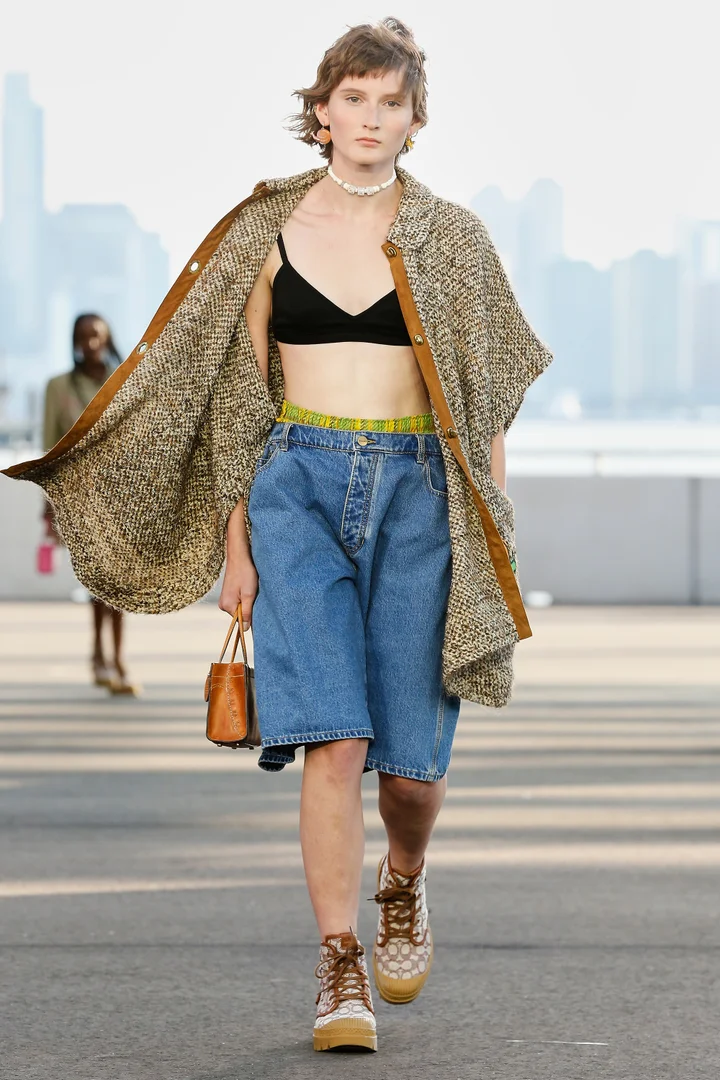The photograph captures a young woman, likely in her late 20s, with very light skin and short brown hair, walking in an urban environment with a hazy skyline and indistinct skyscrapers in the background. She exudes a serious demeanor as she gazes at the camera. Her outfit is a blend of casual and chic: she dons a white collar necklace, vibrant orange earrings, a black bra, and baggy denim shorts that reach her knees. Over her ensemble, she wears a light brown, cream-colored short-sleeve coat or buttoned shirt. Her footwear consists of beige sneakers or booties with brown shoelaces. In her right hand, she gracefully holds a small tan leather purse. Her overall look is completed with a poised, runway-ready presence, suggesting she might be modeling summer fashion in a public setting.